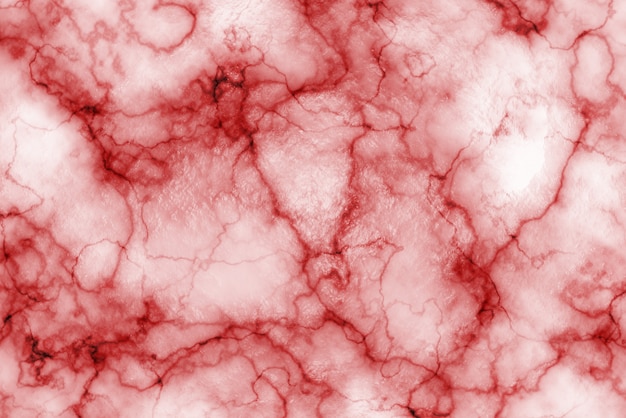The image is a photographic close-up of a surface resembling red and white marble or possibly magnified tissue of a living organism. It features a chaotic and intricate pattern of squiggly and wiggly lines intersecting throughout, creating a dynamic, almost vein-like appearance. These lines vary in shade from dark red to lighter red and pink, often outlined by a faint pink hue. The background is predominantly lighter, with swirls of reds, pinks, and whites mixing together, making it difficult to pinpoint a clear focus. Dense networks of lines suggest veins or blood vessels, with some leading into sections that resemble cell-like structures. The overall image, rectangular in orientation, is devoid of any text or figures and captures the detailed and segmented yet unstructured nature of the composition.